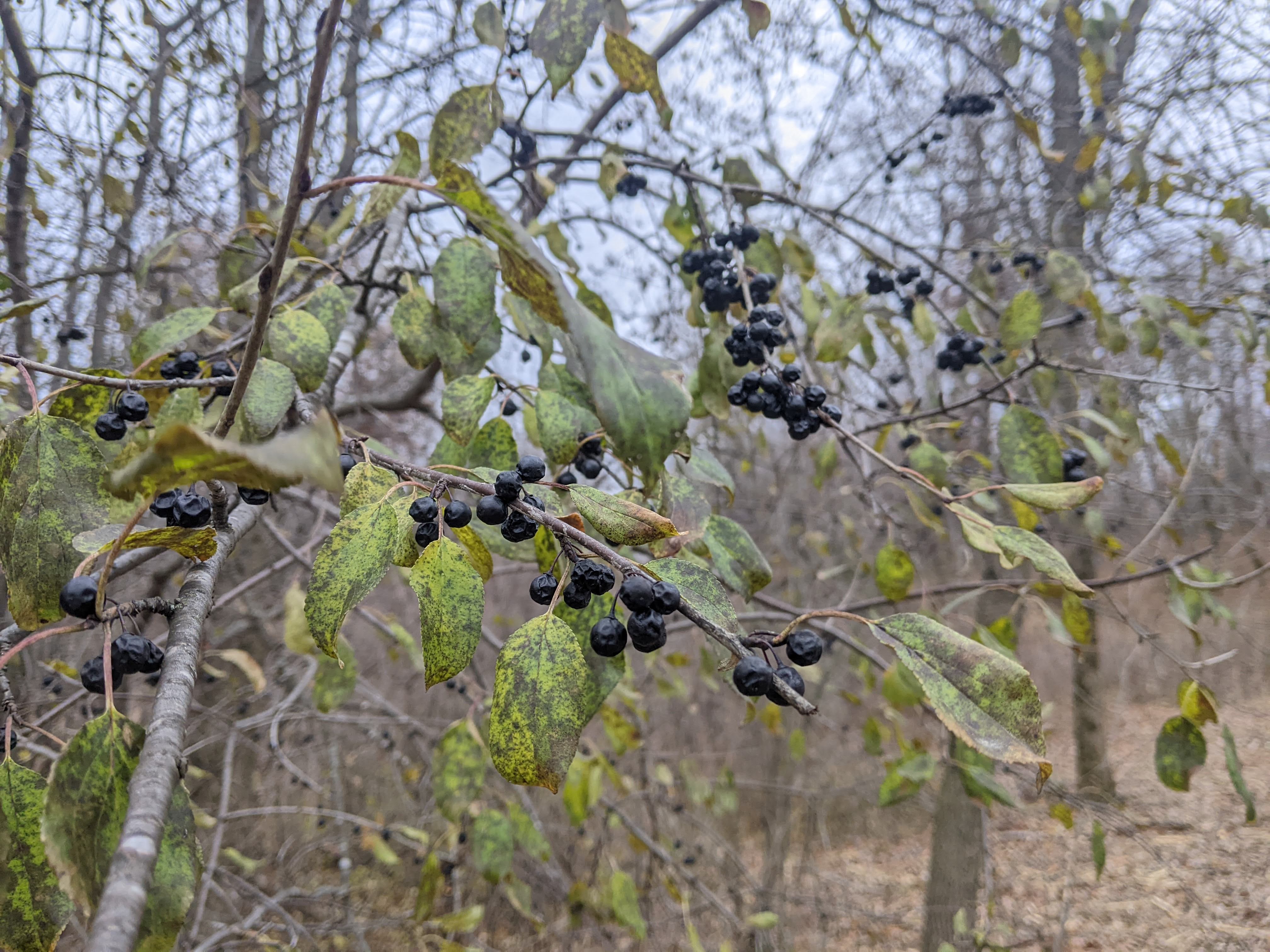The photograph captures a detailed foreground of a shrub or small tree, likely a chokecherry or serviceberry, with smooth gray and white bark. The primary focus is on the shriveling black berries clinging to thin, scraggly branches. These berries, previously round and plump like blueberries, have dried up, suggesting possible drought or disease. Accompanying the berries, the leaves have turned from green to a mottled yellow and brown, with many appearing ready to fall. In the blurred background, bare undergrowth and sparse, leafless trees suggest a distressed environment. The ground is covered in brown, dried leaves and lacks any greenery, further emphasizing the dryness and degradation of the area. The overall effect is one of a dying or struggling plant amidst an arid, neglected landscape.